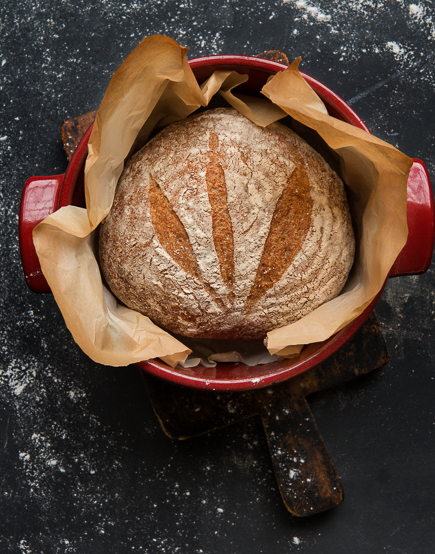This is an overhead photograph of a kitchen setup featuring a freshly baked loaf of bread. The main element is a red porcelain dish with handles on either side, placed on a dark wooden cutting board. The board sits on a black kitchen countertop, lightly dusted with white flour. In the center of the image is a round loaf of bread, resting inside the dish on a piece of now tan-colored parchment paper. The bread is dusted with white flour, and features three distinct slits on top, which have opened up during baking to reveal a light brown crumb beneath the darker crust. The overall composition and details emphasize the artisanal quality of the bread and the rustic kitchen environment.